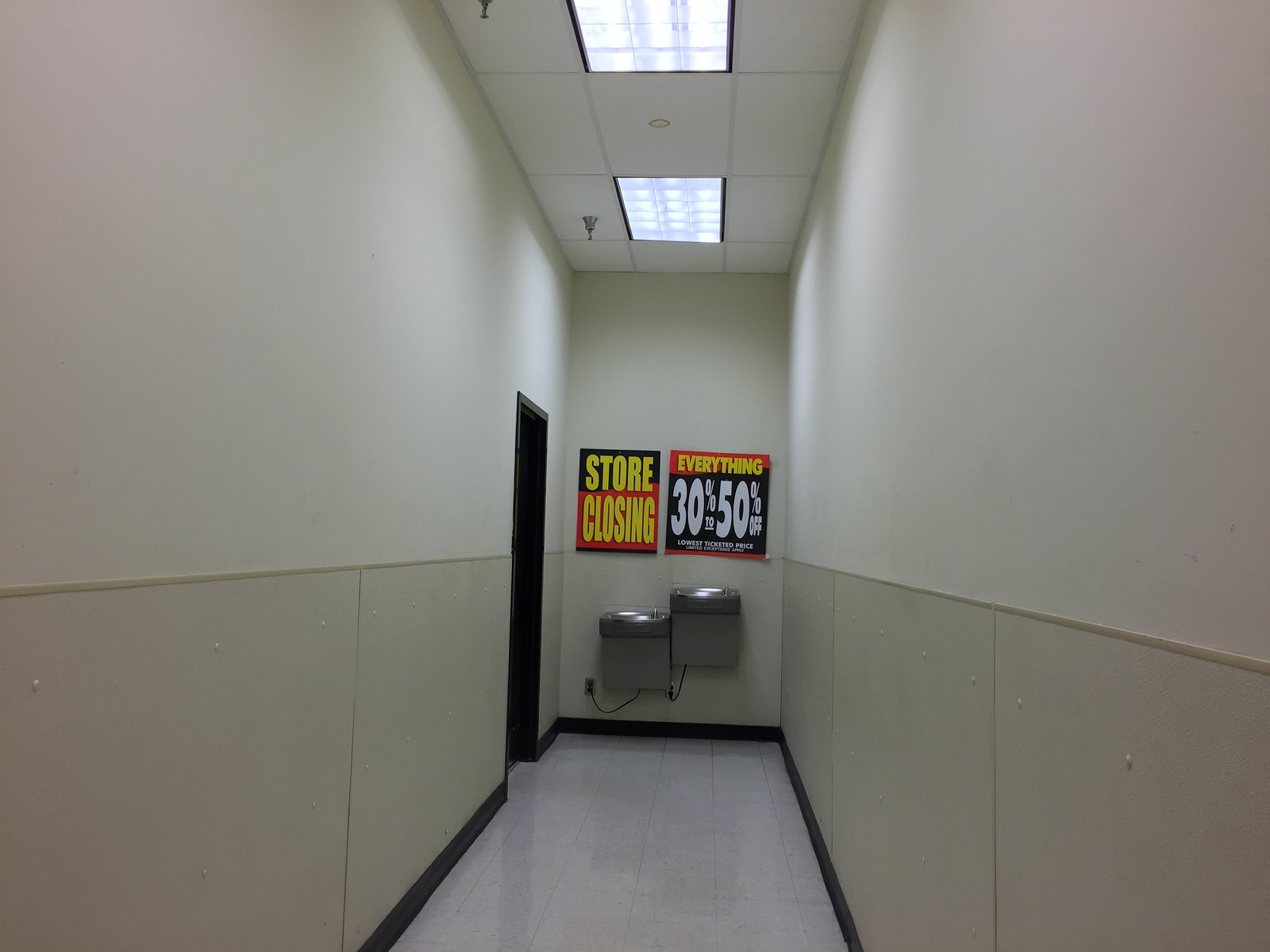This is a detailed photo of a hallway, likely inside a Macy's store, viewed from one end towards the other. The hallway is narrow and has a partial view of the back wall, which is divided into a white upper half and a tan lower half, accentuated by a black baseboard running along the floor. The floor is covered in white tiles, and the ceiling is made up of white fiberboard tiles, housing a large rectangular fluorescent light fixture and a fire sprinkler on the left side.

At the end of the hallway, there is a black door on the left and two water fountains mounted on the wall. These fountains are positioned close to each other but at different heights, with the right one being slightly higher than the left. They are plugged into an electrical outlet located towards the bottom left side of the wall. Above the water fountains, there are two posters on black backgrounds. The left poster displays the message "Store Closing" in large yellow letters, while the right one announces "Everything 30 to 50% Off Storewide" in giant white numbers.